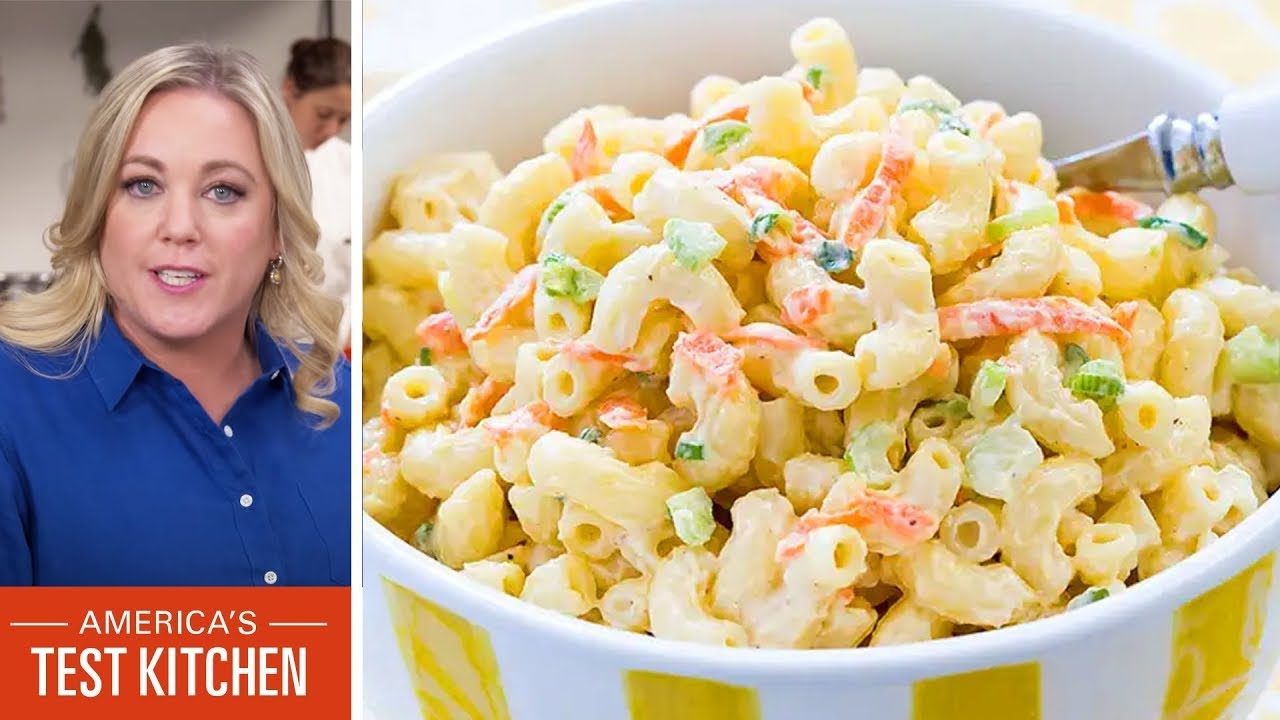This detailed advertisement for America's Test Kitchen features a dual-image layout. The larger image on the right, occupying about two-thirds of the space, showcases a white bowl adorned with thick, horizontal yellow stripes. Inside the bowl is a steaming, cheesy macaroni dish mixed with finely peeled green and orange vegetables, possibly carrots and green onions, creating a vibrant contrast. A silver utensil, its neck partially visible, protrudes from the right side, complemented by a glimpse of its white handle.

On the left side, which takes up roughly one-third of the space, a close-up photo captures a blonde-haired woman with blue eyes, dressed in a dark blue button-up shirt. Her mouth is slightly open, suggesting she’s about to speak. Behind her, another woman with brown hair tied up in a bun can be seen, wearing a white shirt. The background appears to be in a light beige tone. Below this image, an orange rectangular banner with white text prominently reads "America's Test Kitchen," emphasizing the advertisement's brand.